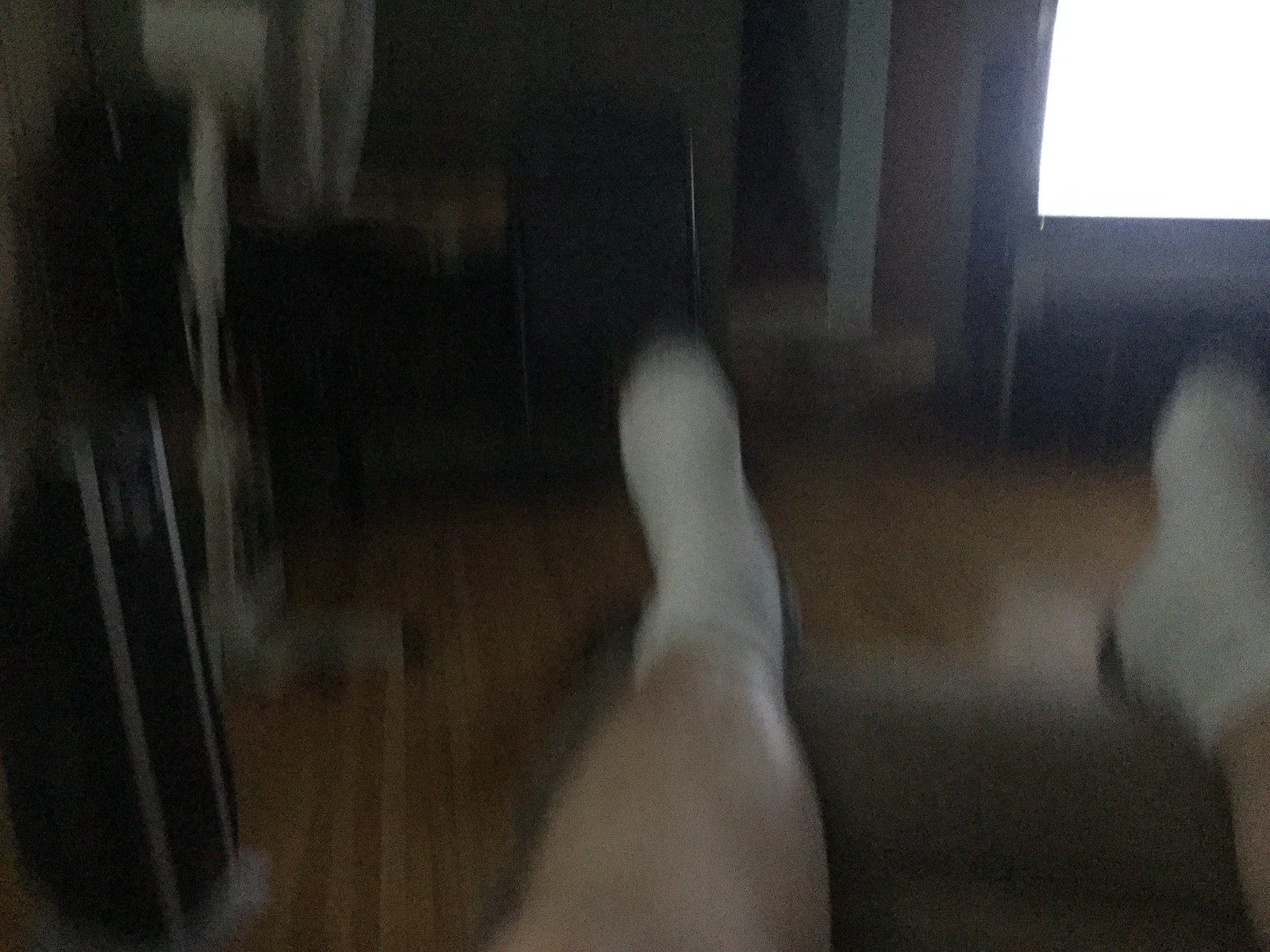The image captures a dimly lit and blurry scene of a larger individual reclining in a chair. The focus is on their legs, which extend from the knee and mid-calf down. The person's legs are clad in white ankle socks, and they have fair skin. Their feet rest on an olive green cushion, suggesting either an ottoman or part of the chair they are using. The setting features a brown wooden floor that adds a rustic touch to the room. Opposite the person, light streams through a window, illuminating part of the space. To the left, a black structure with silver elements is visible, which appears to be either a fan or a space heater, adding a functional aspect to the cozy environment.